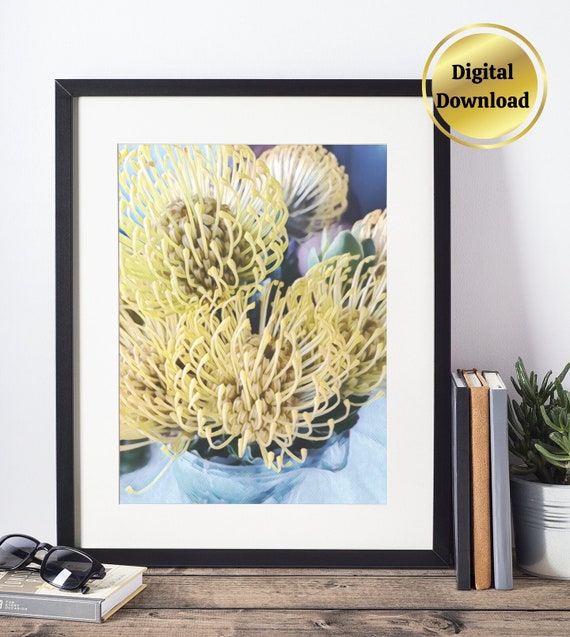This is a photograph depicting a styled console, possibly in a hallway or entryway of a home. In the top right corner, a gold circle with the words "Digital Download" signifies this image may be available for purchase as stock content. The main focus of the composition is a framed floral picture leaning against the wall. The artwork, encased in a black frame and bordered by white canvas, showcases a close-up of vibrant yellow flowers in a pot, with a hint of blue hues in the background.

The scene is adorned with additional elements on the wooden shelf. To the left of the framed picture lies a book positioned flat with an unreadable title, topped with a pair of black sunglasses. To the right, three nondescript books stand upright beside a white ceramic pot housing a green cactus-like plant. The arrangement of these items gives off a casual, beachy vibe, making the setting appear cozy and inviting. The overall design suggests the photograph could be used as a decorative stock image for websites or other projects needing a touch of home decor elegance.